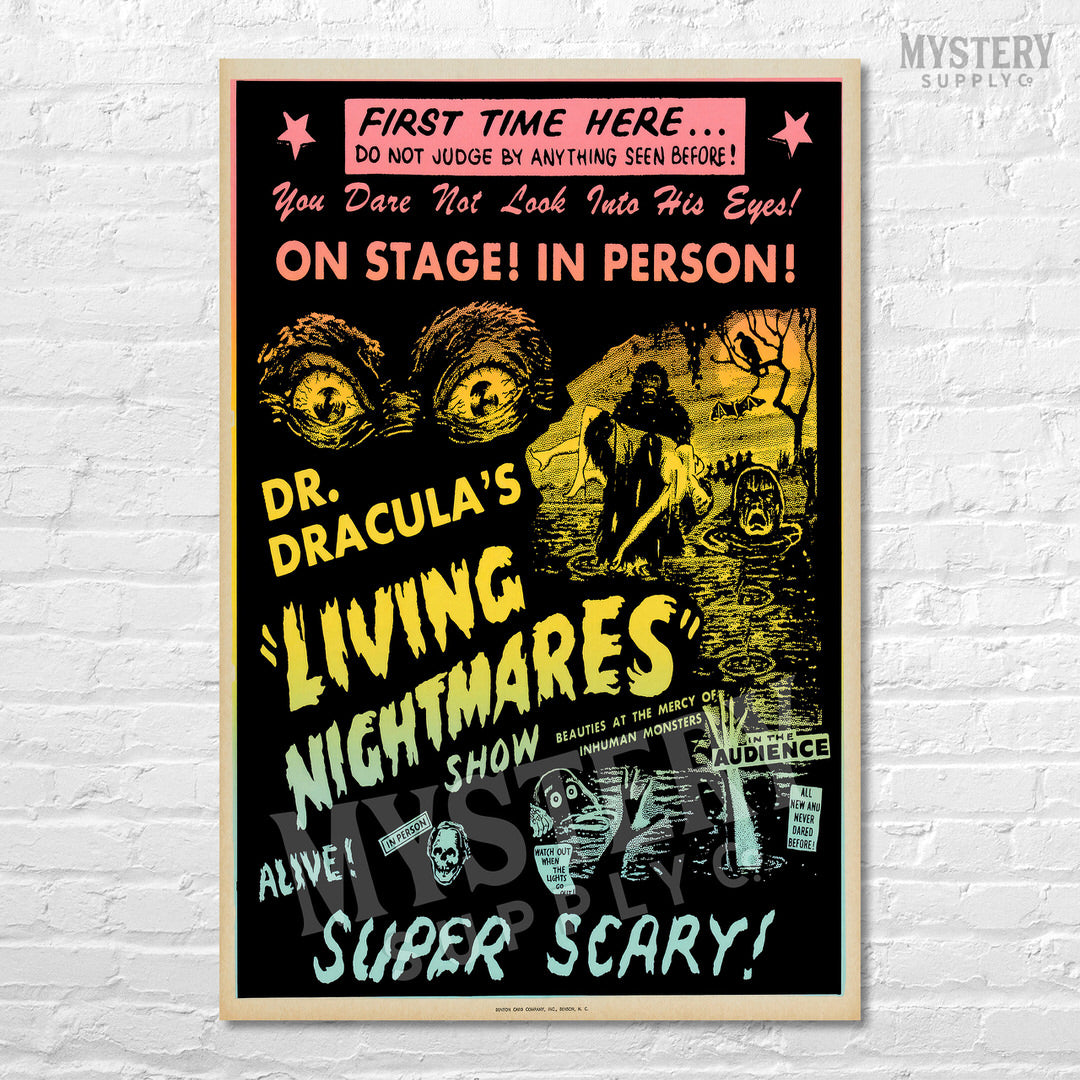The image showcases a photoshopped poster on a white wall with visible thin, rectangular bricks. The poster, outlined by a thin, tannish light brown border, has a black background. At the top, a light red rectangle is flanked by red stars on either side. Below this, in a cursive red text, it reads, "You dare not look into his eyes." The next section, set against a light pink background, announces in black letters, "First time here, do not judge by anything seen before!" 

Further down, "You dare not look into his eyes, on stage, in person," is written in a light peach-orange color. Underneath, in yellow text, it boldly advertises "Dr. Dracula's Living Nightmares Show" and declares in blue letters, "Alive and super scary." Accompanying this text are vivid images: two yellow, gorilla-like eyes staring ominously, a gorilla carrying an unconscious woman, a creature's head emerging from a lagoon, a vulture perched on a bare-branched tree, and a bat flying overhead. Towards the bottom, it warns of "Alive beauties at the mercy of inhuman monsters" and cautions "Watch out when the lights go out," promising an experience "All new and never dared before."